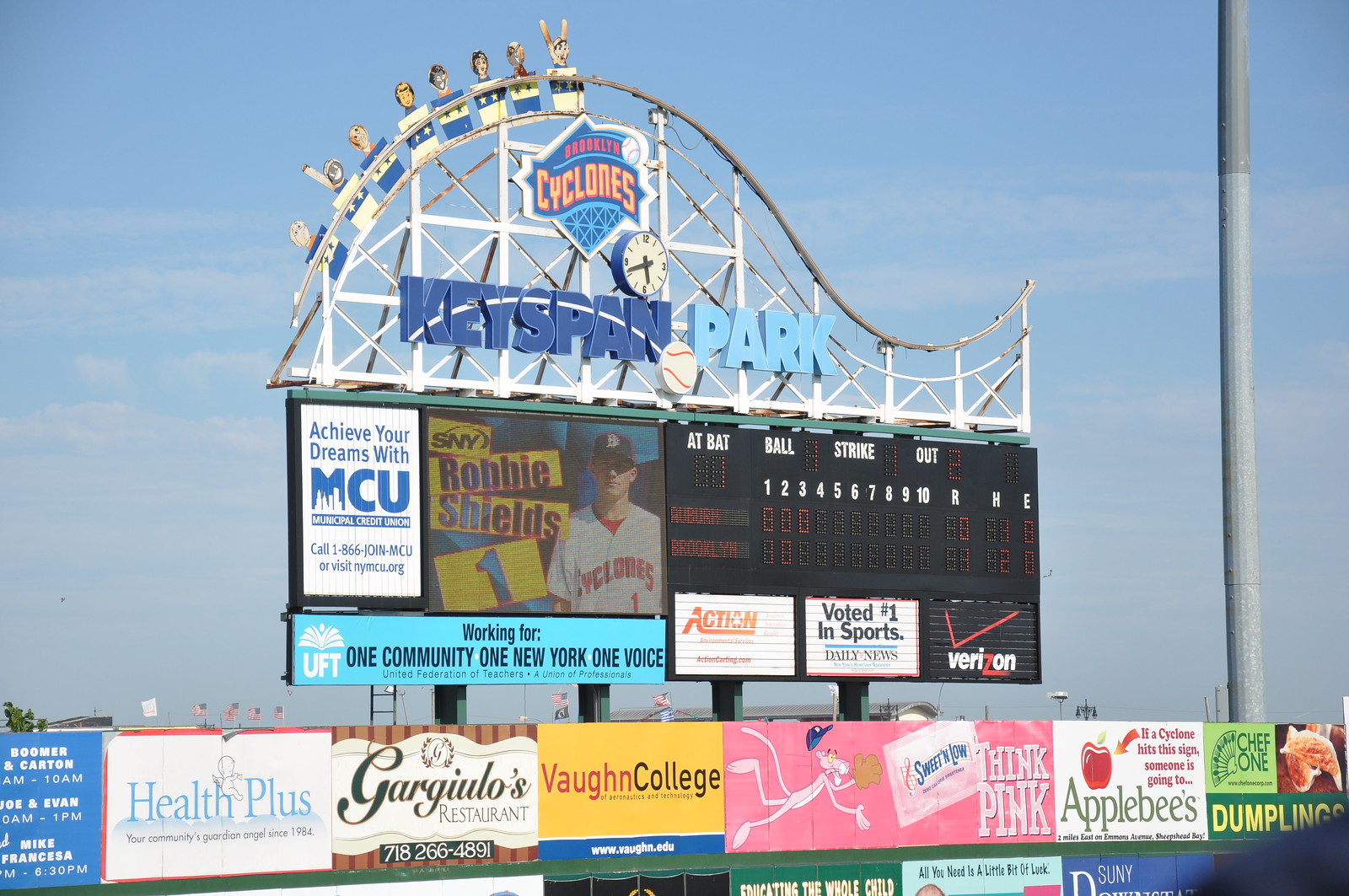The image depicts a vibrant scene at KeySpan Park, a minor league baseball stadium in New York. Dominating the foreground is a large, ornate scoreboard framed by a beautiful blue sky. The top of the scoreboard features a whimsical, stylized depiction of a rollercoaster with animated sketches of children riding the cars. Above this rollercoaster illustration, the words "Brooklyn Cyclones" are prominently displayed. Centrally located on the sign is a large clock, reading approximately 5:40 PM. Below the clock, in bold capital letters, the words "KeySpan Park" are split into navy blue "KEYSPAN" and light blue "PARK."

Further down, the scoreboard includes various signs and advertisements. One part of the board highlights Robbie Shields with the phrase "Achieve Your Dreams with MCU" and "Working for one community, one New York, one voice." Another section details the game information, listing at-bats, balls, strikes, and outs, with placeholders for scores yet to be filled.

A range of advertisements occupies the bottom tier of the sign, including promotions for Verizon, the Daily News, UFT, Sweet 'n Low, Applebee’s, Health Plus, Gargiola's Restaurant, and Vaughan College. In front of this towering scoreboard is a traditional outfield wall lined with additional signage, completing the bustling, sponsor-rich atmosphere characteristic of a minor league ballpark. The scene encapsulates the lively, communal spirit of a beautiful day at the ballpark, inviting fans to enjoy the game amidst a sea of colorful advertisements and playful art.